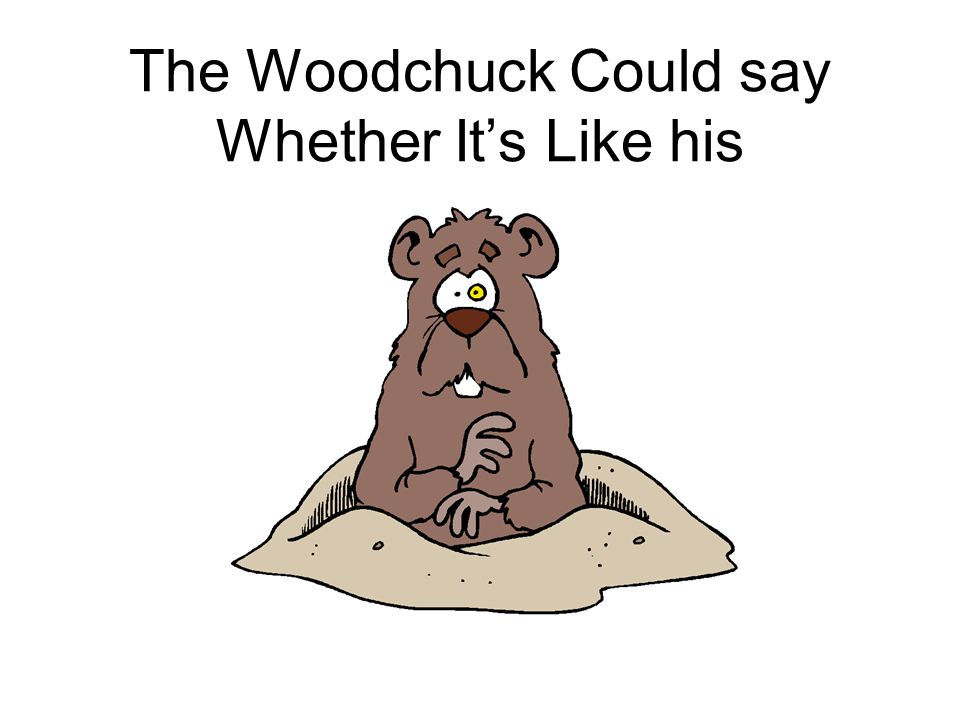This is a detailed cartoon drawing of a woodchuck emerging from a mound of dirt against a white background. The woodchuck is light pastel brown with darker brown accents on its nose and eyebrows. It features two distinctive eyes: the left eye is noticeably larger with a yellow circle around the pupil, while the right eye is smaller and solid black. This gives it an appearance that might suggest curiosity or surprise. The woodchuck has small buck teeth protruding from its mouth and holds its lighter brown hands in front of its body, conveying a sense of anxiousness. The creature's round ears are set atop its head, and the black text above it reads, "the woodchuck could say whether it's like his," arranged on two centered lines. This illustration is likely a scanned image, possibly from a children's book, given its digital coloring and whimsical style.